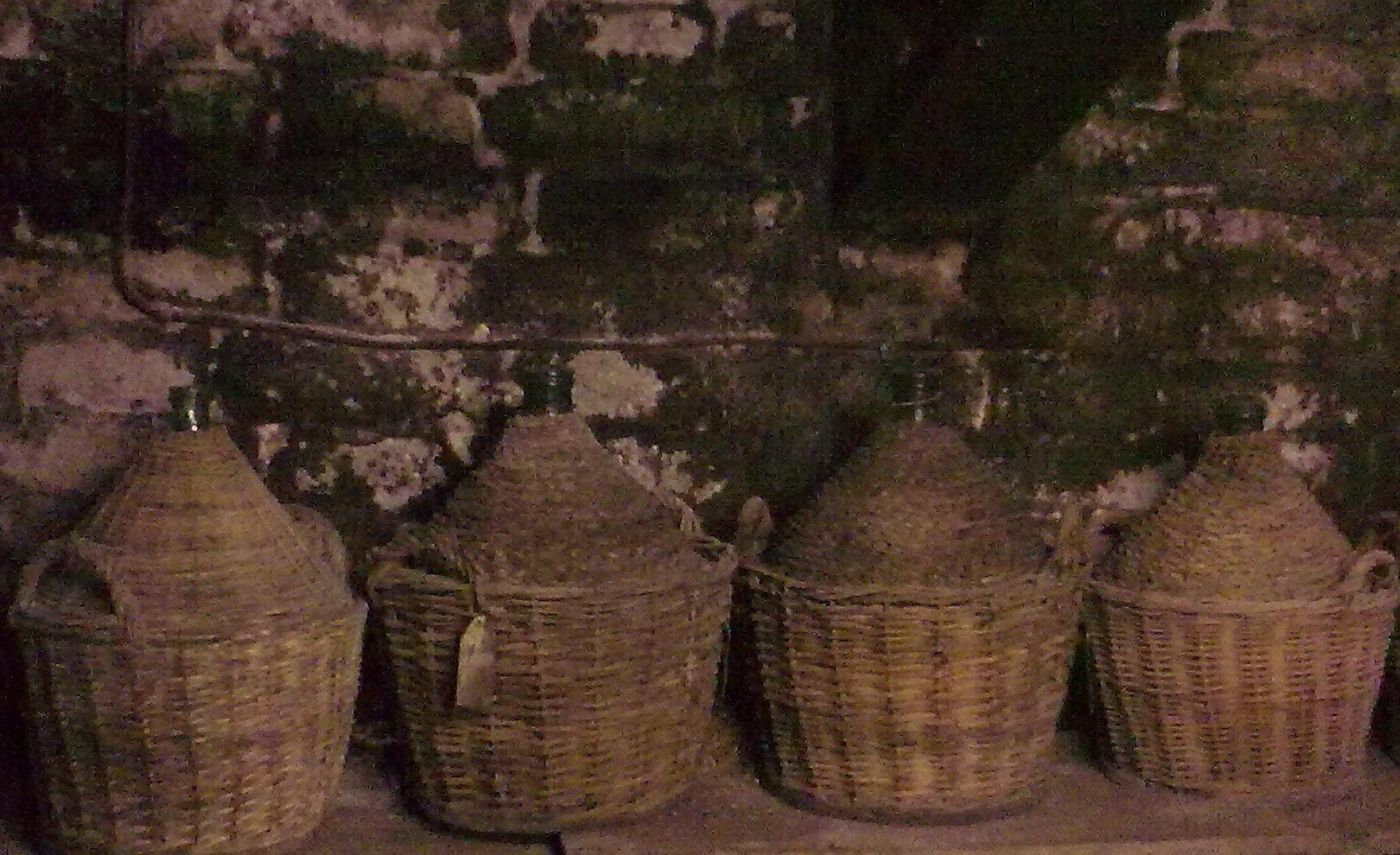The image depicts four cylindrical wicker baskets, likely made of rattan or raffia, arranged in a row on a sandy or dirt-covered ground. Each basket features two upside-down U-shaped handles and is topped with a conical lid that encloses a greenish bottle, giving the baskets a pointed appearance at the top. The second basket from the left has a distinct golden tag attached to its handle. The background features a moldy and decrepit cinder block wall with patches of darker brown and white, indicating wear and tear. Visible along the wall is a horizontal pipe that makes an L-shaped bend on the left side of the image, possibly made of aged copper or silver. In the upper right-hand corner, a dark beam protrudes from the wall, adding to the rustic and deteriorating ambiance of the scene.